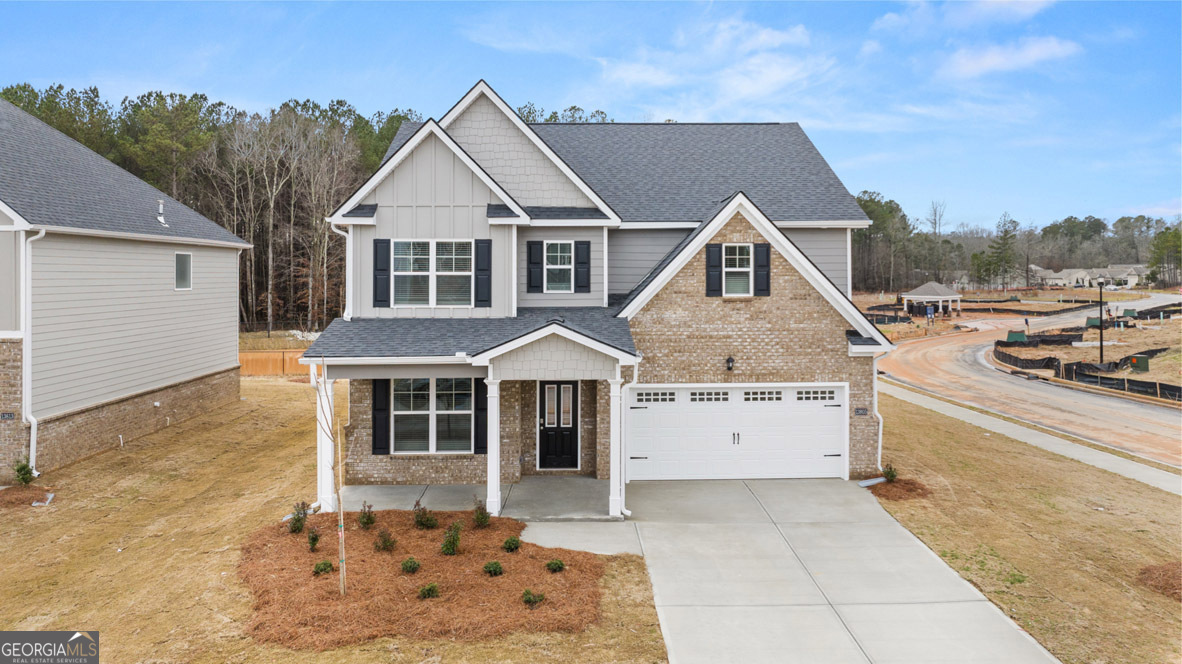The image showcases a newly completed two-story house in a developing neighborhood. The house features a light brown and white brick front, complemented by sections of light gray to blue wooden siding, and a dark gray roof. It has three windows on the upper floor, a large window on the lower floor, and a door with two small windows. The house includes a white two-car garage with a light above it. Dark gray shutters frame the windows. The landscape around the house includes patches of brown grass, small newly planted bushes, pine straw, and a young tree without leaves, indicating it is winter.

The neighborhood appears to be in an early stage of development, with additional houses and construction visible in the background. Tall deciduous trees, some green and others leafless, populate the horizon under a bright, clear sky with light blue tones and minimal white clouds. A glimpse of urban sprawl and planned green spaces can be seen, suggesting an effort to blend suburban development with natural elements.